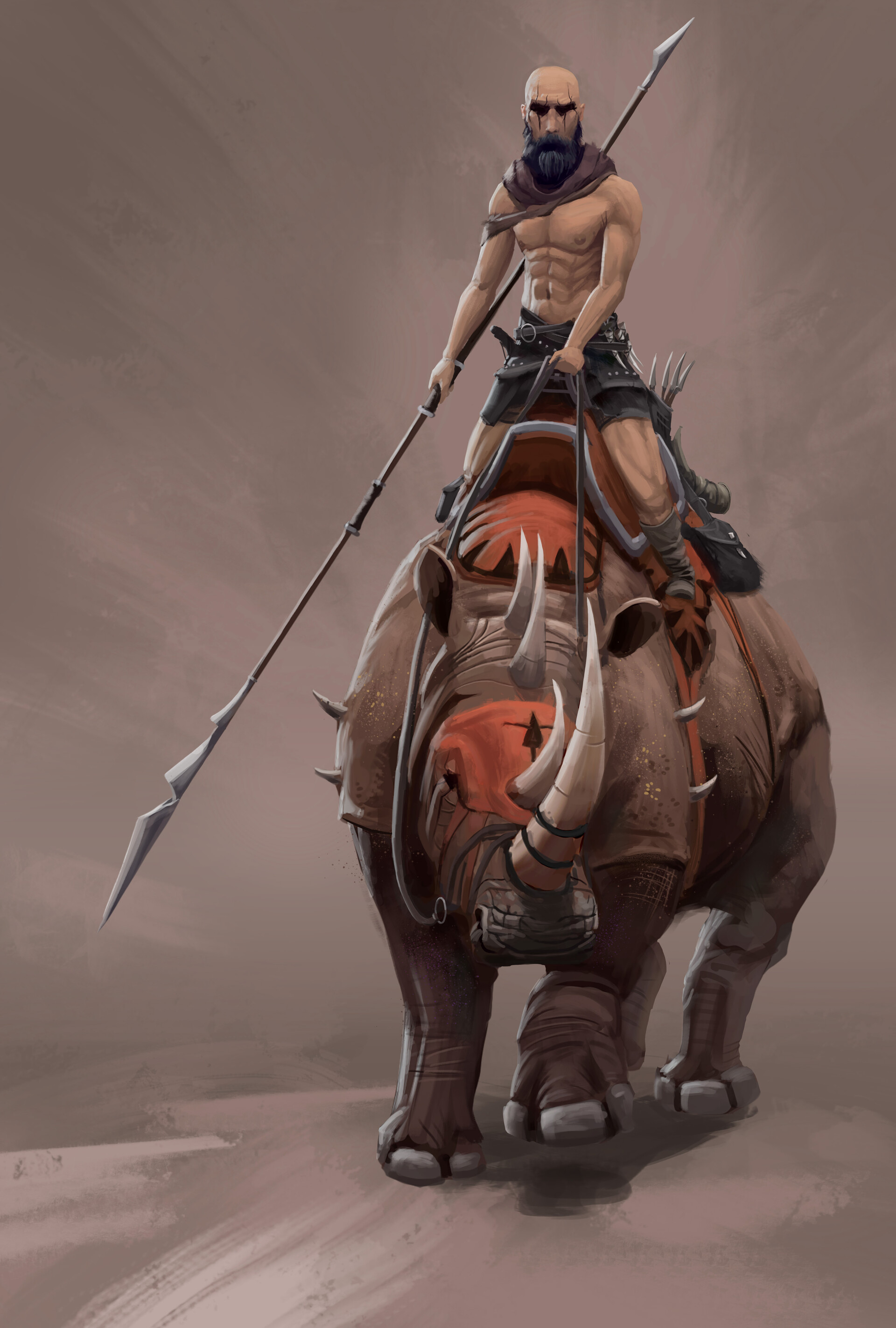This fantasy art drawing depicts a muscular, shirtless, bald man with brown skin, wearing only black shorts and a black scarf around his neck, sitting on a heavily armored grey rhinoceros. Holding a long, pointed spear, estimated to be around 12 feet long, in his right hand, the man guides the rhinoceros with reins held in his left hand. The rhinoceros, adorned with an orange protective band around its nose and greyish body, is facing the viewer with four prominent tusks—two long white horns protruding from its snout and two shorter ones on its head. Its left front hoof is lifted as though walking. The saddle on the rhinoceros is detailed in orange and black, flanked by menacing spikes on either side. The background consists of a smoky, blurry grayish hue that adds an air of mystery and adventure to the scene. The contrast of the gray ground, streaked with white, enhances the dramatic, action-packed ambiance of the image.